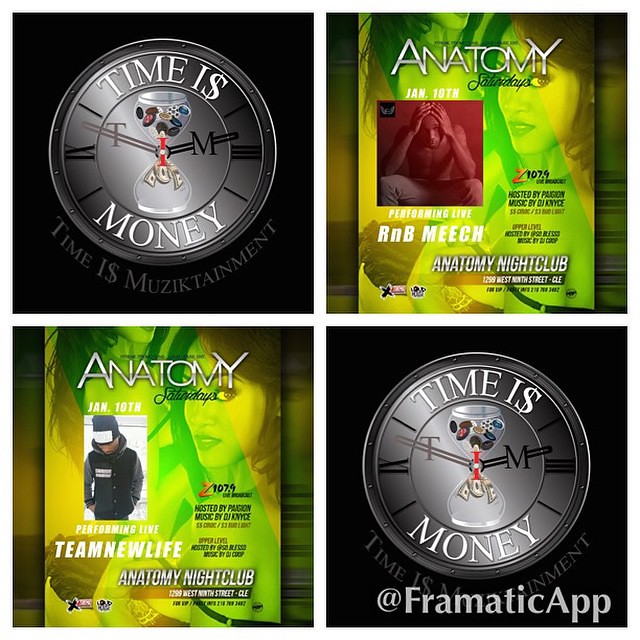This image is a photo collage consisting of four equally-sized panels. The top-left and bottom-right panels are identical, showcasing a logo on a black background resembling a watch interface. Centered on the logo is the phrase "Time is Money," with the 'S' in 'is' stylized as a dollar sign. An hourglass is depicted within the logo, with clock hands pointing to around 2:48. 

The other two panels, positioned diagonally from each other, feature almost identical magazine covers titled "Anatomy Saturdays" with the tagline "Z 107.4." However, they differ slightly in content. One cover highlights a Black African American male with the caption "Performing Live: R&B Meech," and the other features a different Black African American male with the caption "Performed Live: Team New Life." Both magazine sections also mention "Anatomy Nightclub."